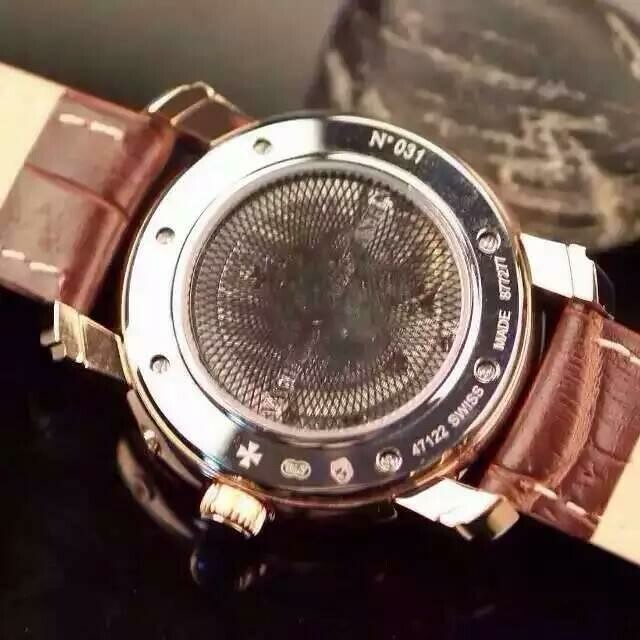This detailed photograph captures the intricacies of the back side of a silver watch. The close-up image shows the watch's winder prominently positioned towards the bottom of the frame. Notable features include the number '31' printed clearly on the back and a Swiss cross decoration directly opposite. The words 'Swiss Made' are etched into the surface, flanked by the numbers '47122' on one side and '877277' on the other. The watch is secured with a robust leather strap in a ruddy brown tone, accentuated with beige stitching. The scene is set against a dark surface that appears to be a black or gray table, providing a stark contrast that highlights the watch's details.